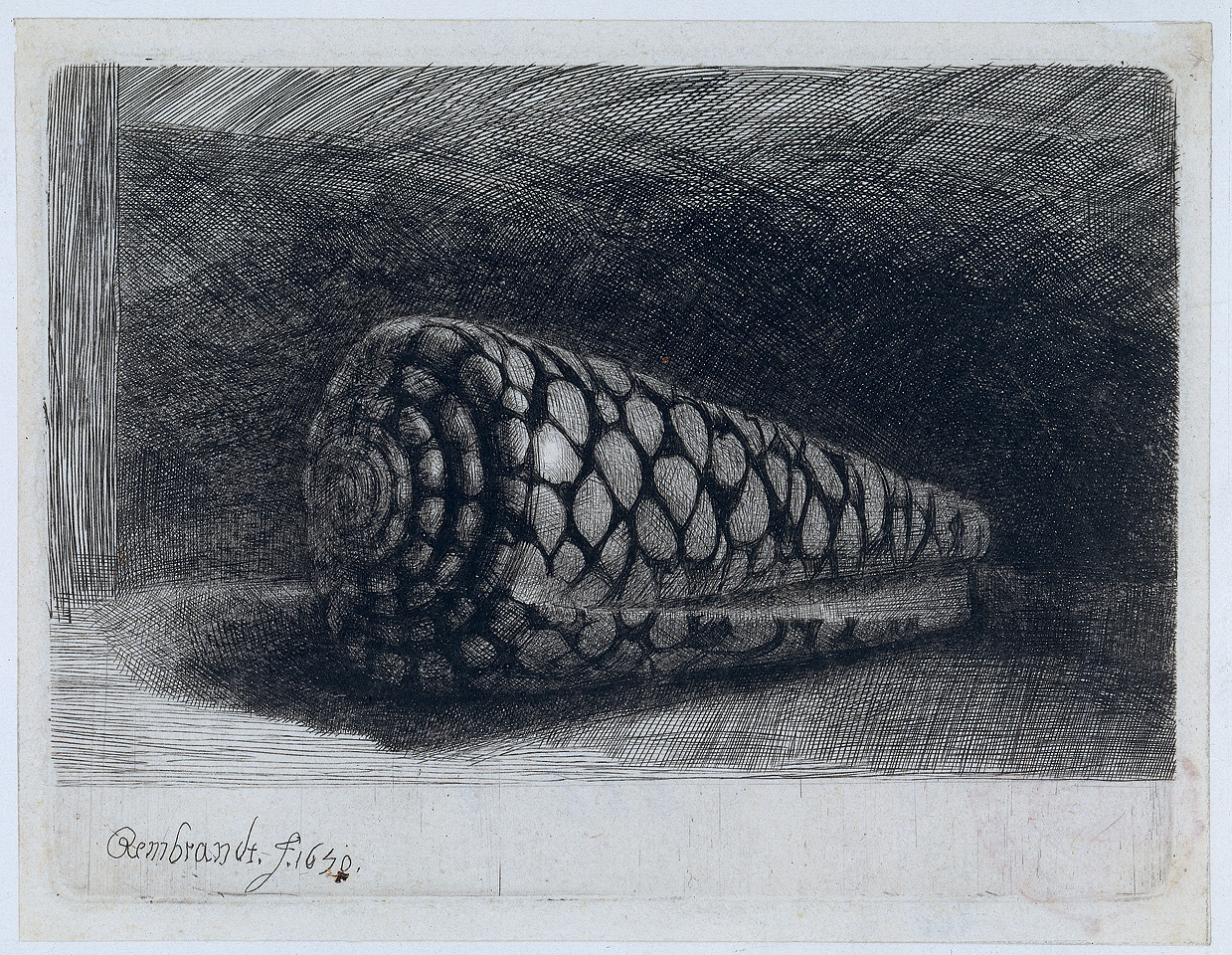This black and white image, a detailed hatch drawing possibly by Rembrandt from 1650, presents a complex scene of intersecting thin black lines. The centerpiece of the image shows a singular rolled object resembling a pine cone or an old rolled-up carpet with intricate designs. The drawing is characterized by numerous white spots separated by these black lines, giving the object a textured appearance that evokes a river of stones when unrolled. Positioned diagonally, the object extends from a thicker foreground on the left to a thinner background on the right, creating a sense of depth. The image appears to be bordered by an off-white or light gray frame, adding contrast to the expressive strokes. In the drawing's bottom left corner, a possible signature of Rembrandt is faintly visible. The background consists of darker and lighter hatchings and thin squiggly lines that might represent wood graining, adding to the depth and detail of this remarkable artwork.